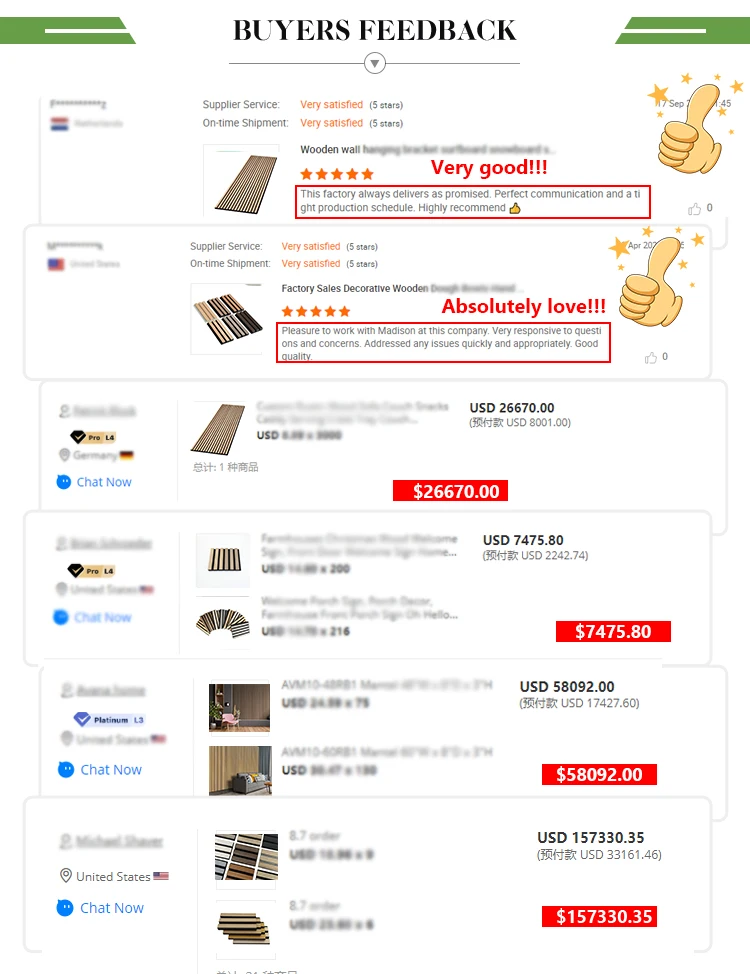The webpage features a section titled "Buyer's Feedback," displaying a series of review boxes. Each box showcases feedback on a supplier's service, with ratings indicating "Very Satisfied" for aspects like service quality and on-time shipment, accompanied by a five-star rating system. The primary product discussed is a wooden wall hanger bracket, though much of the content regarding it is blurred. Positive testimonials highlight the factory's reliability, effective communication, and adherence to tight production schedules, concluding with a "Highly Recommend" endorsement and a thumbs-up icon.

The next highlighted review underlines the factory's sales of decorative wood, with most of the details obscured. It mentions a positive experience working with Madison from the company, noting her responsiveness and efficiency in addressing questions and concerns, ultimately rating the quality of the product favorably and giving another thumbs-up.

Below these detailed reviews, the page includes four additional blurred-out ads or listings, presumably related to different wooden products. The listed prices are $26,670, $7,475, $58,992, and $157,330.35, respectively. The context suggests that the webpage belongs to a company dealing in a variety of wood products, showcasing customer satisfaction and product offerings.